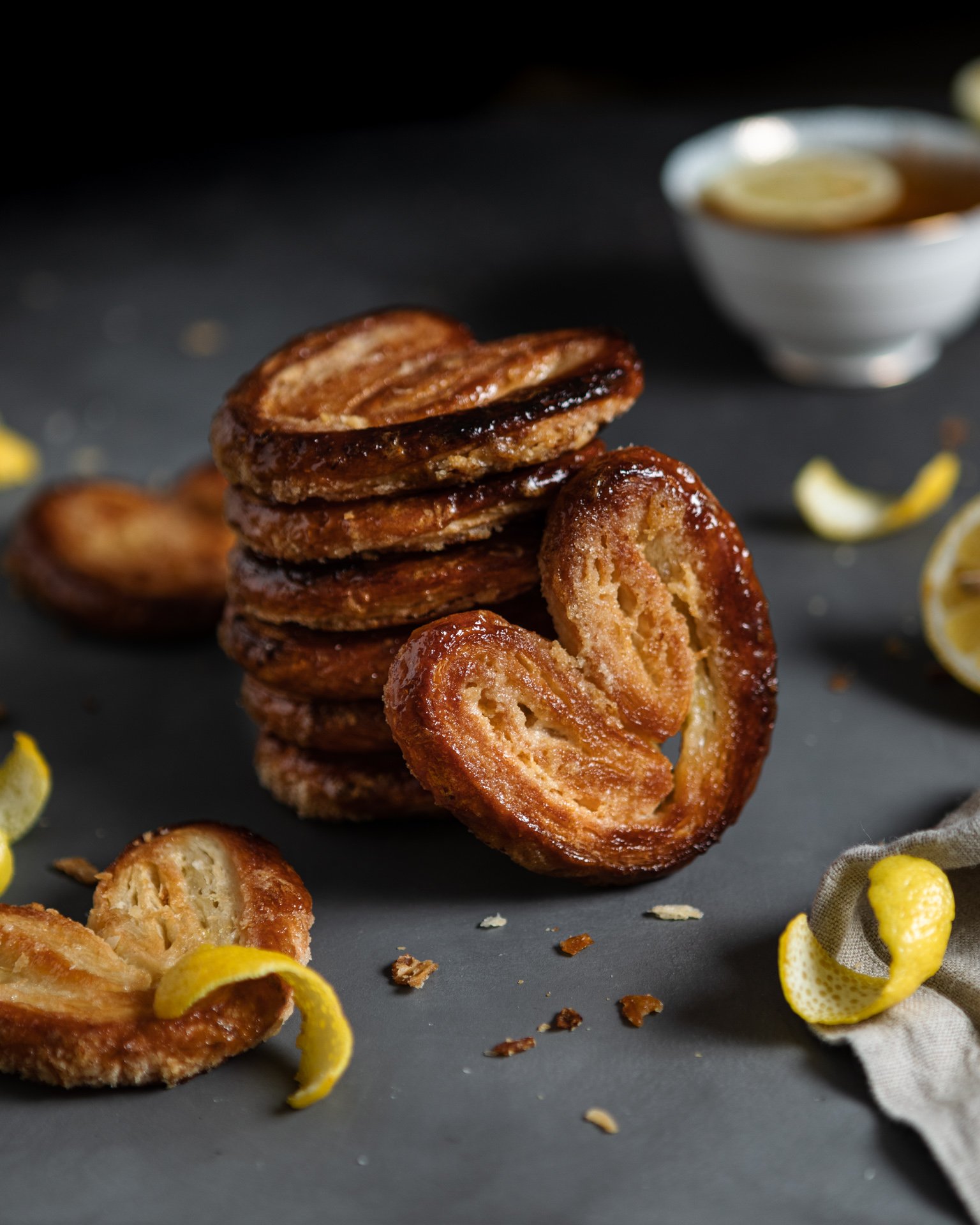This photograph, taken indoors, showcases a delightful arrangement of freshly baked heart-shaped pastries, commonly referred to as palmieres or elephant ears. These pastries, made from glossy puff pastry, are arranged in a stack of six on a gray countertop, reaching about 2 inches high. One pastry leans against the stack on its most visible side, while another lies flat beside it. Scattered around the scene are slices and curls of lemon rind, adding a touch of zest to the composition. In the upper right-hand corner of the image, there is a delicate white teacup with a gold rim, filled with brown tea and garnished with a thin slice of lemon. A white kitchen towel peeks into the frame from the bottom right corner, completing the cozy, culinary setting. The top portion of the photograph is slightly blurred, drawing focus to the central display of heart-shaped pastries.